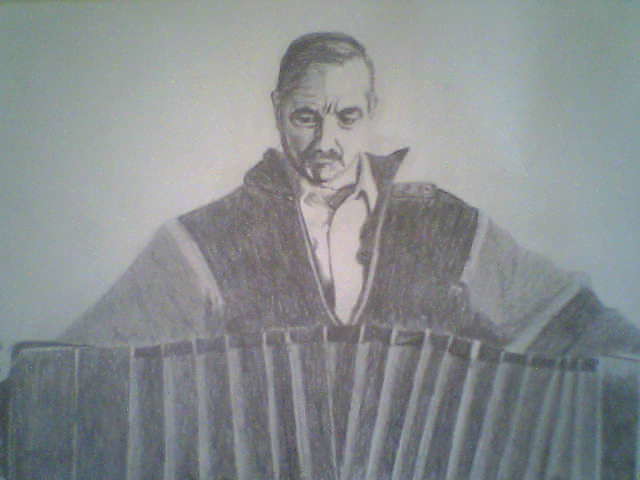The image depicts a man with a distinctly vampiric appearance, sporting deep wrinkles on his face, especially noticeable between the eyes. His short, dark hair frames strikingly black eyebrows and a prominent black mustache. He wears a high-collared, vampire-like cape paired with a buttoned-up, lighter-colored shirt that appears to be in an off-white or slightly more vibrant tone. The artwork seems to be a meticulously drawn black and white sketch, possibly done with pencil, charcoal, or colored pencils, lending a textured, hand-crafted look to it. The background is white, providing a stark contrast to the figure standing centrally. Adding to the detail, the man is in front of a curtain, and the foreground features a segmented black mortar-like object or perhaps a sectioned sand arena. The collar and sleeves of the cape are particularly notable, with the sleeves having a mid-section that is off-white and a darker-colored bottom portion.